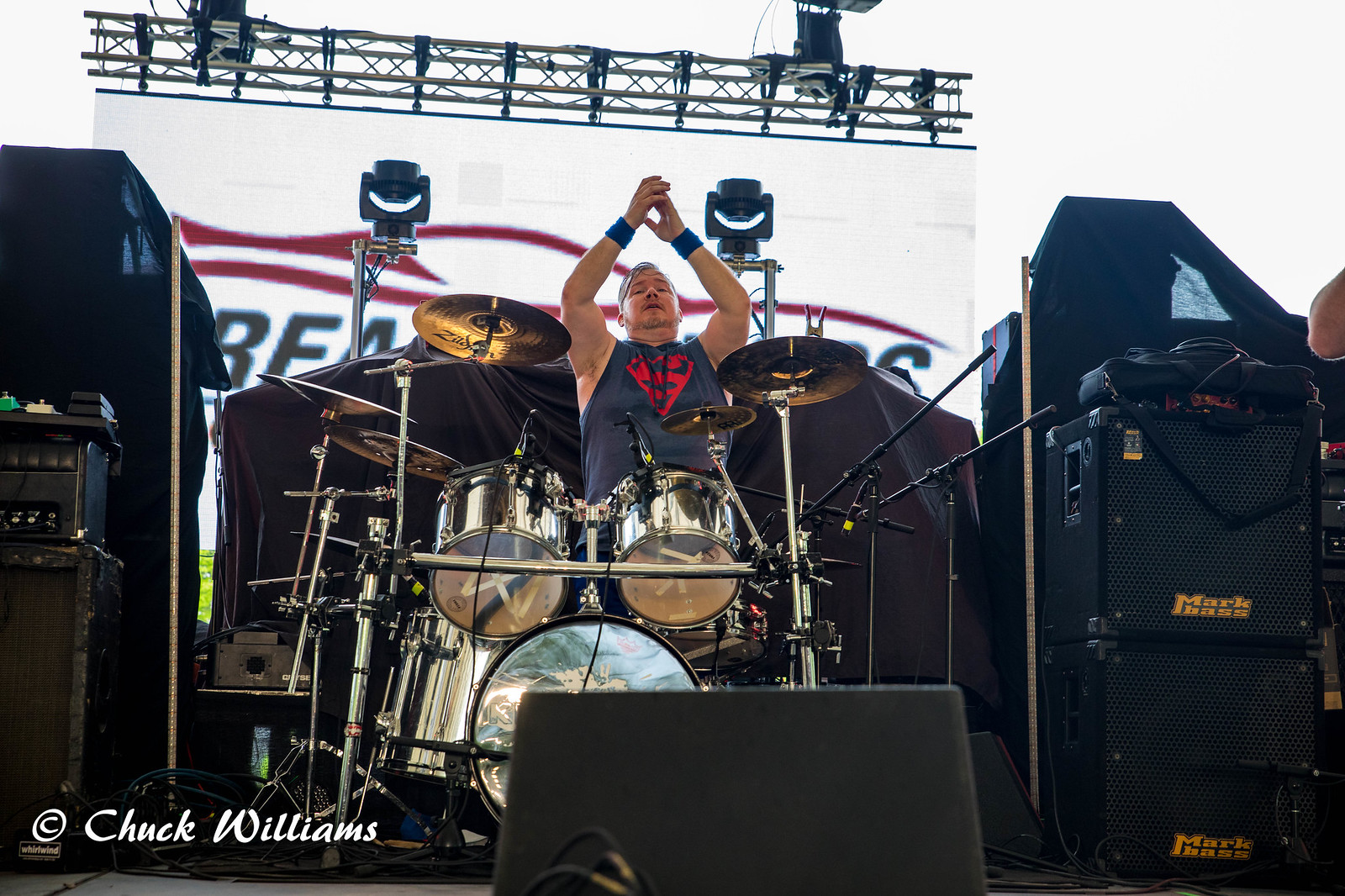This outdoor concert photograph, taken by Chuck Williams, captures a dynamic moment on stage featuring a drummer behind a silver drum set adorned with Zildjian cymbals. The drummer, dressed in a distinctive red suit and a black tank top featuring a red Superman logo, raises his hands above his head as if encouraging the audience to clap along. His wrists are adorned with sweatbands, and there are notable details such as a stage rig with lights overhead and various amplifiers flanking him. To the left, a guitar amp and a cabinet are partially obscured by a black cloth, while to the right, there are two stacked Mark Bass bass cabinets. There is a backdrop with a partially legible logo starting with "BE" on the left side. The bright, possibly white sky above suggests the event is outdoors, and a white sign hangs in the background from a steel beam. Additionally, the lower left of the photograph contains the photo credit and copyright information: "Copyright Chuck Williams."